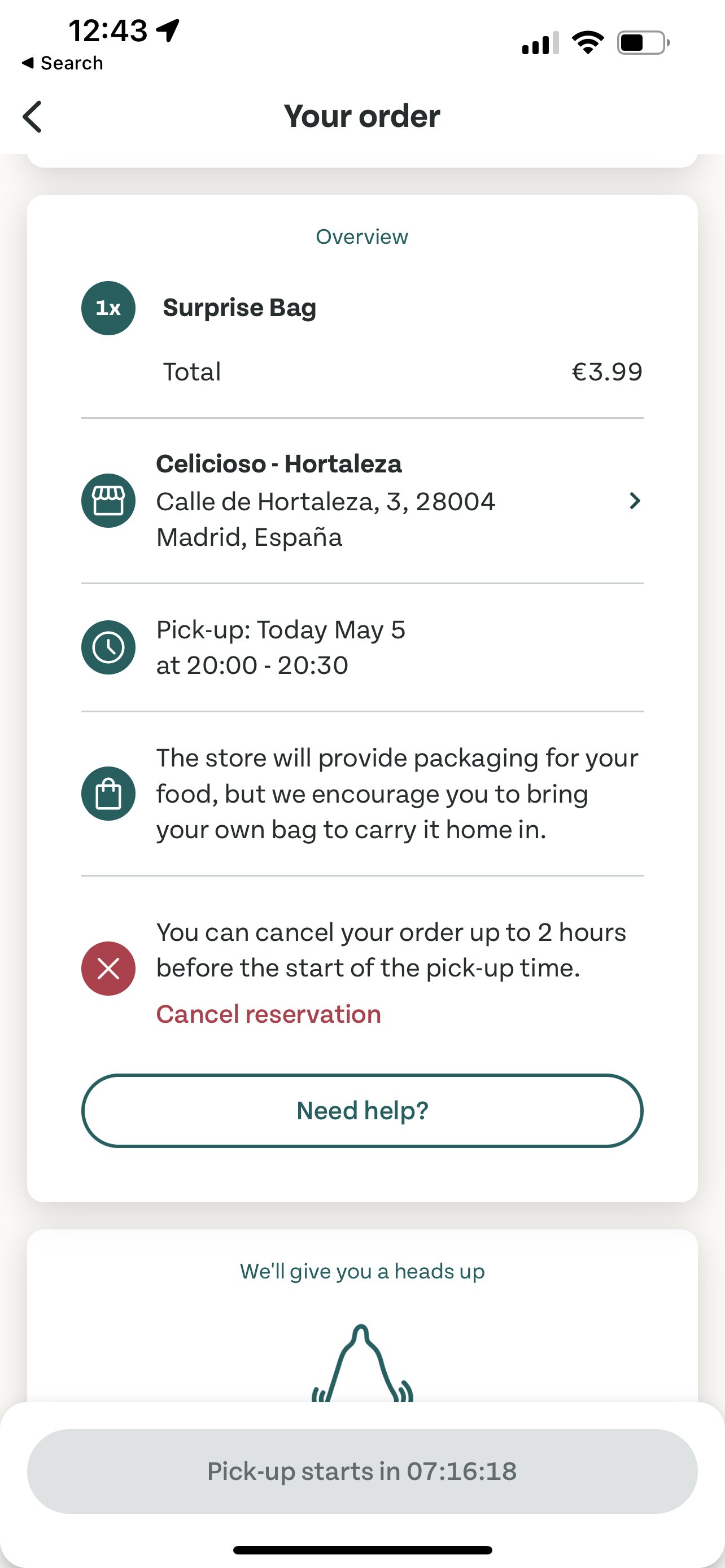At 12:43, the screen displays an order summary with various system notifications: location services are enabled, there are 3 out of 4 signal bars, full Wi-Fi connectivity, and the battery is at half capacity. The top center of the screen reads "Your Order." Below is an overview showing that a "One-Time Surprise Bag" totaling 3.99 euros has been ordered from Selesioso located at Calle de Hortaleza, 328-004 Madrid, España. The pickup is set for today, May 5th, between 20:00 and 20:30. The store will provide packaging but recommends bringing a personal bag for carrying the food home. Additionally, a red circle highlights that the order can be canceled up to 2 hours before the pickup time. There are options to "Cancel Reservation" and a "Need Help" section. A grey oval at the bottom indicates, "Pick-up starts in 07:16:18," with a black section at the very bottom confirming the details.